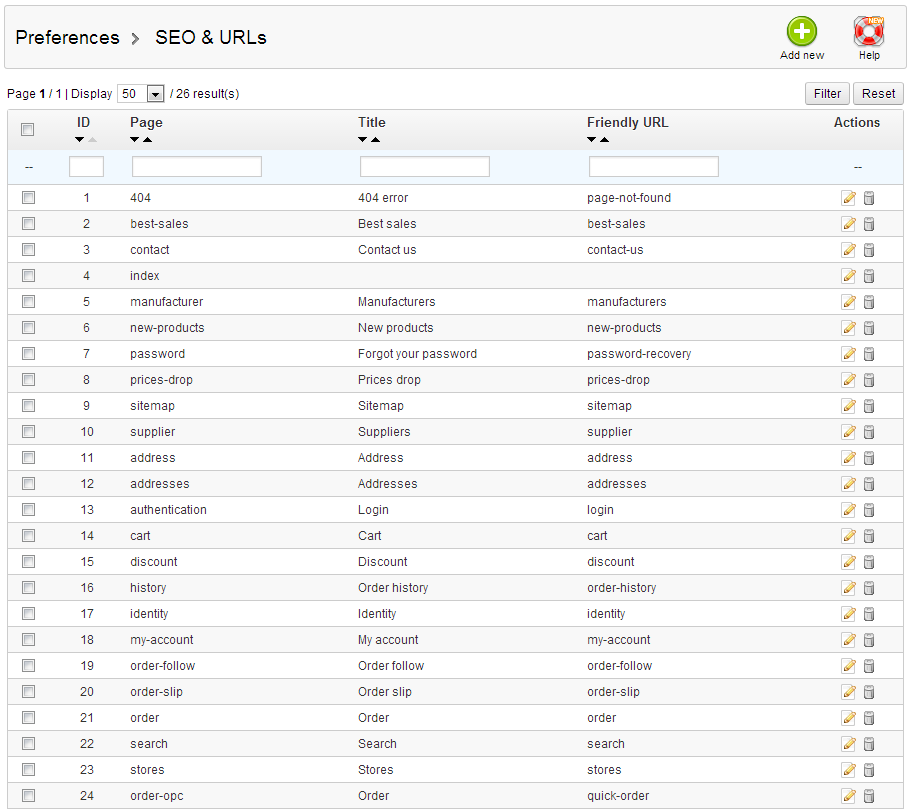In this image, we see a detailed interface displaying a list of settings or records on a white background. The layout is structured with various rows of information presented in horizontal lines, organized in a vertical stack for easy readability.

At the very top, there's a header that reads "Preferences, SEOs, and URLs". Just below this header, there's a control panel displaying "Page 1 of 1" and "Display 50", with the number 50 inside a drop-down box, indicating the number of entries displayed per page.

Following this, the main content area is divided into 24 distinct lines or rows, each containing specific information. Each row includes fields for ID, Page, Title, Friendly URL, and Actions. For instance:

1. The first row (ID 404) lists a page labeled "404", with the title "404 error" and the friendly URL "Page Not Found".
2. The second row (ID 2) displays "Best Sales" as the page, title, and friendly URL.
3. The third row (ID 3) has the page labeled "Contact", the title "Contact Us", and the friendly URL "Contact Us".
4. The fourth row (ID 4) is labeled "Index" but lacks both a title and a friendly URL.
5. The fifth row (ID unspecified) shows "Manufacturer" as the page, with both the title and friendly URL set to "Manufacturers".

This pattern continues down to the bottom of the list, with various entries following a similar format but containing different data for each record. The interface appears to be a management tool for organizing and editing website URLs, titles, and other related preferences.